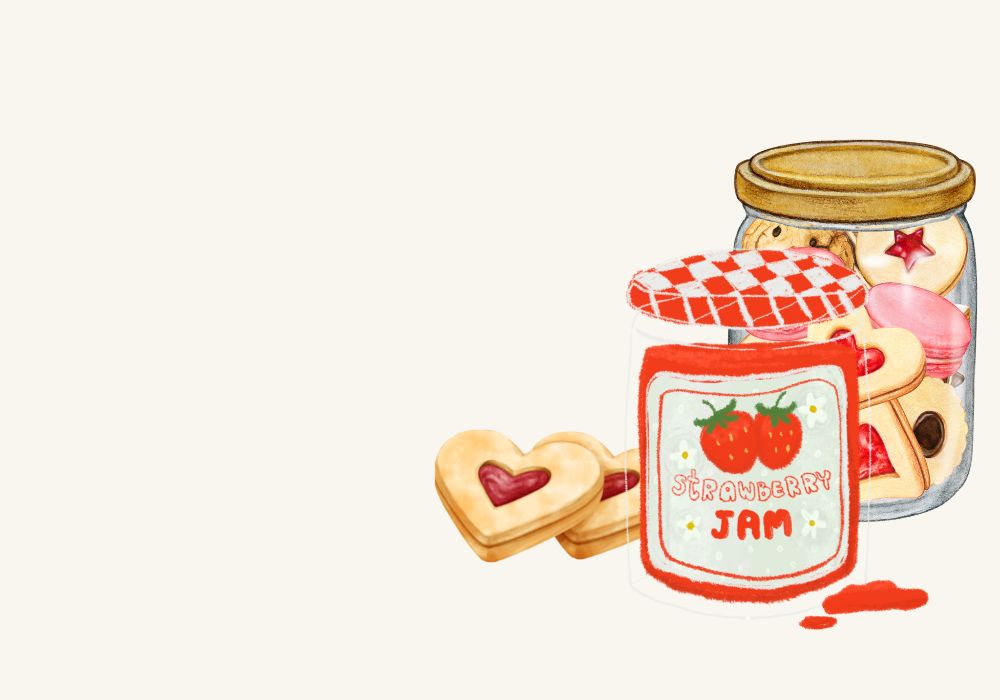This image is a detailed drawing of cookies and strawberry jam set against a white background. The left side of the image is entirely empty, highlighting the focus on the elements concentrated on the right side. The main subject is a clear glass jar of strawberry jam in the foreground, adorned with a red and white checkered lid. The jar features a painted label with two strawberries at the top, and the words "strawberry" in white and "jam" in red, encircled by a red stripe. Adjacent to this jar are two heart-shaped cookies with light brown exteriors and strawberry jam-filled cut-out centers, revealing their delicious filling. To the right is a second glass jar with a wooden lid, filled with an assortment of cookies; some have red heart and star shapes, while others are pink meringue cookies. The upper left corner of the image is clear, except for a small area where red jam is dripping, enhancing the visual appeal. The image beautifully captures the essence of a sweet, homemade treat scene.